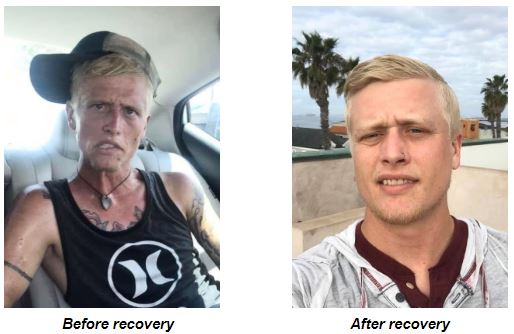The image is a pair of color photographs arranged on a white background, displaying a before-and-after comparison of a man who went through recovery. Both photographs are labeled, with the left image captioned "before recovery" and the right image captioned "after recovery." 

In the "before recovery" image on the left, the man is sitting in the backseat of a white car. He has pale skin, straggly blonde hair, and a sharp jawline. He wears a dirty black and white baseball cap turned sideways, a black sleeveless top with a white circular X logo, and a necklace. His body and neck are adorned with tattoos. His facial expression is unpleasant, with a slight frown and mouth slightly open, and he appears quite ill and haggard.

The "after recovery" image on the right shows the same man in an outdoor setting near the seaside, with palm trees and small buildings in the background under sunlight. His hair is neat and clean, and he has a fuller, healthier appearance with a slight smile. He is wearing a burgundy shirt with a hoodie. Overall, the man looks much healthier and content in the "after recovery" image, providing a stark contrast to his earlier appearance.